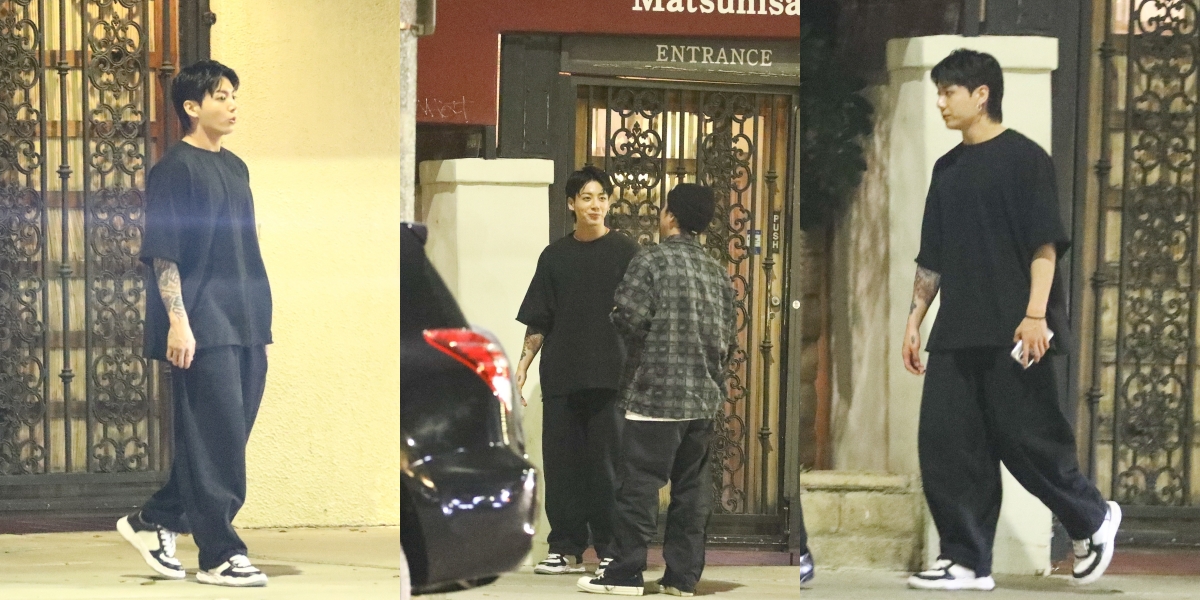In this outdoor photograph, there are four young gentlemen, likely in their mid-teens, with an iron design covering the doors and windows in the backdrop, which may indicate the entrance to a restaurant named "Matsumsa" as suggested by the signage. Two of the individuals are walking on a primary sidewalk, facing each other. The young man on the left is dressed in a blue sweatpants suit. Opposite him, walking towards the left, another young man in a black sweatsuit with white sneakers accented in black holds a rectangular white object in his left hand and displays tattoos from his elbow to near his wrist on his right forearm.

In the background, two more teenagers are interacting. One wears a plaid-style shirt paired with black bottoms and black sneakers with white accents, while speaking to a young man dressed in a solid black outfit. These interactions occur amid the clear identifiers of the location, such as an iron gate and a prominent "ENTRANCE" sign.

Overall, the setting exudes a sense of everyday life and social interaction among these young men, surrounded by an urban environment with definitive architectural features.